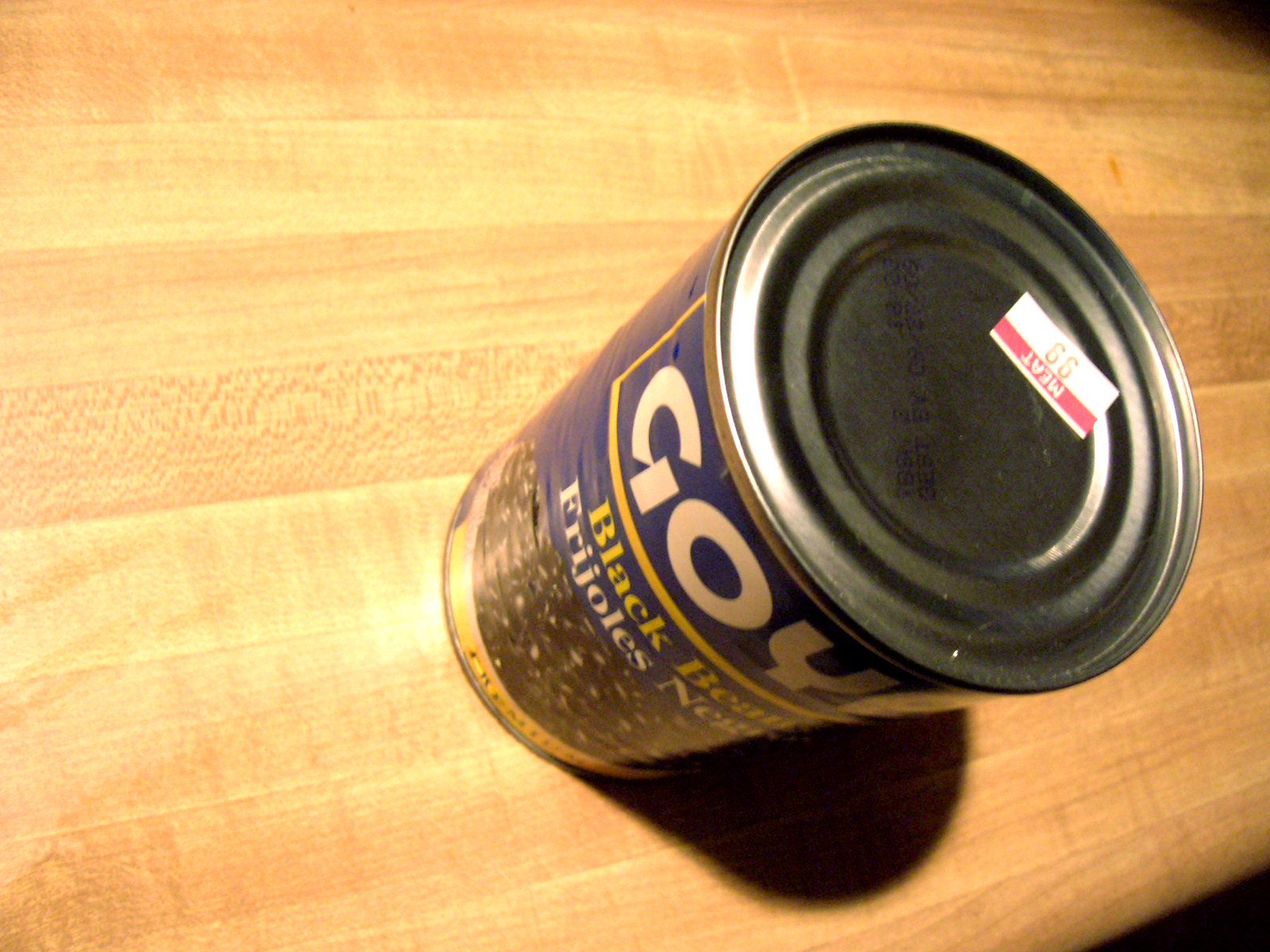In this image, we see a can of food prominently placed on a light-colored wooden countertop or tabletop. The can itself is labeled with a blue and yellow design and features an image of beans on the front. The brand name "Goya" is printed in bold white text, and "Black Beans" is indicated below it in yellow letters. The photograph is taken from a top-down angle, clearly showcasing the can and its details. At the top of the can, there's a price tag that intriguingly reads "meat" and indicates a price of 99 cents. The composition and clarity of the image highlight the product effectively against the neutral background of the wooden surface.